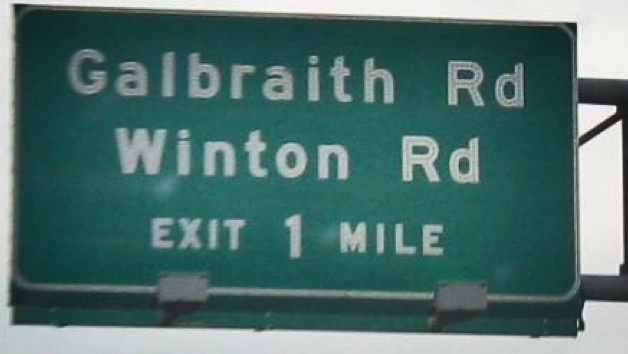This photograph captures an interstate road sign under overcast skies. The sign, a standard green type commonly seen on highways, indicates an upcoming exit for Galbraith Road and Winton Road, located one mile ahead. The text on the sign reads "Galbraith Road" and "Winton Road," with the exit distance clearly marked. Two rectangular lights are mounted to illuminate the sign, although they are turned off due to the daytime setting. The sky is overcast, casting a dull light over the scene, which, combined with the lack of focus and presence of visual artifacts, results in a slightly blurry image. This road sign, occupying the majority of the frame, dominates an otherwise sparse and indistinct background.